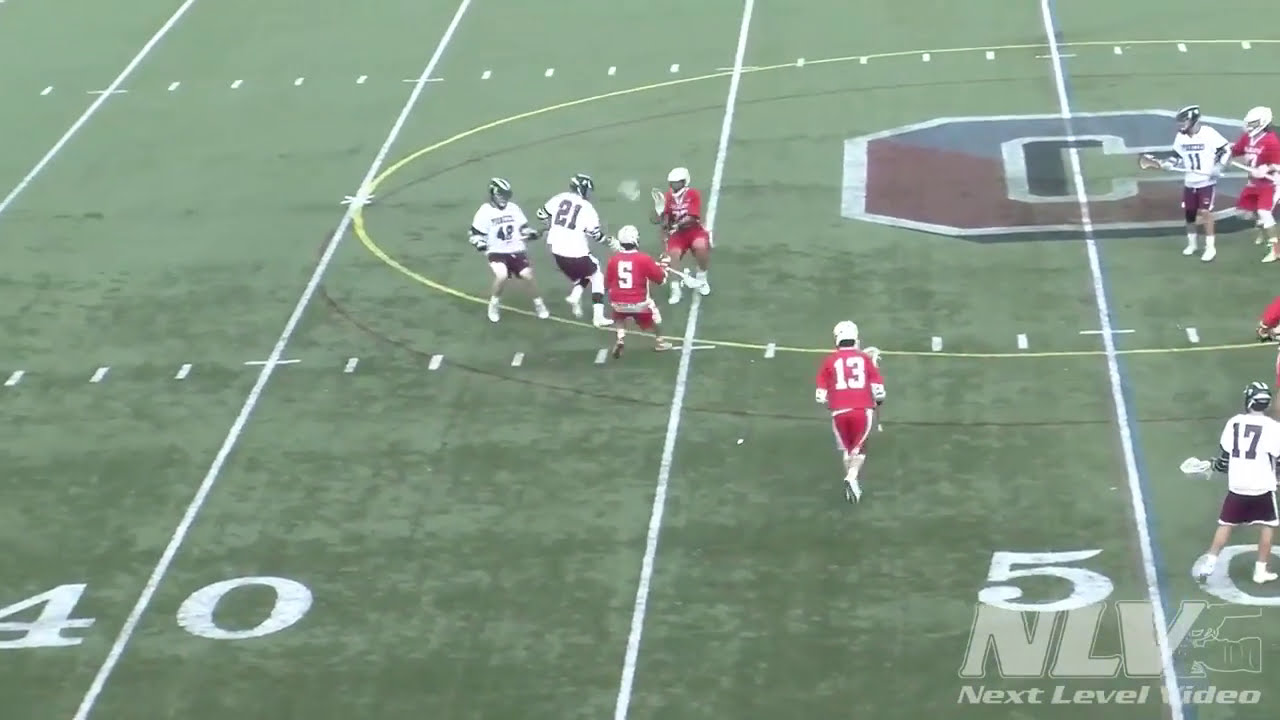The image depicts an intense lacrosse match being played on a green, multi-purpose field marked with football yard lines, specifically between the 40 and 50-yard lines. The game is broadcasted by Next Level Video, as indicated by the NLV logo at the bottom right of the image. Prominently featured in the middle of the field is a large red "C" logo, presumably representing Cornell University's insignia. Eight players are visible on the field; four are wearing white jerseys with black helmets and four are in red jerseys with white helmets. The players' numbers in white jerseys include 42, 21, 17, and 11, while in the red jerseys, numbers 5 and 13 can be seen clearly. The players are equipped with lacrosse sticks and protective gear, including shorts and helmets. Notably, one player in a red jersey, number 5, is on his knees in the middle of a dynamic play, swatting at the ball alongside his teammates and opponents. To his left, players in white jerseys numbered 21 and 42 are engaging in the action. Additionally, player number 17 in a white jersey is seen in front of the "C" logo, holding their stick at hip level.